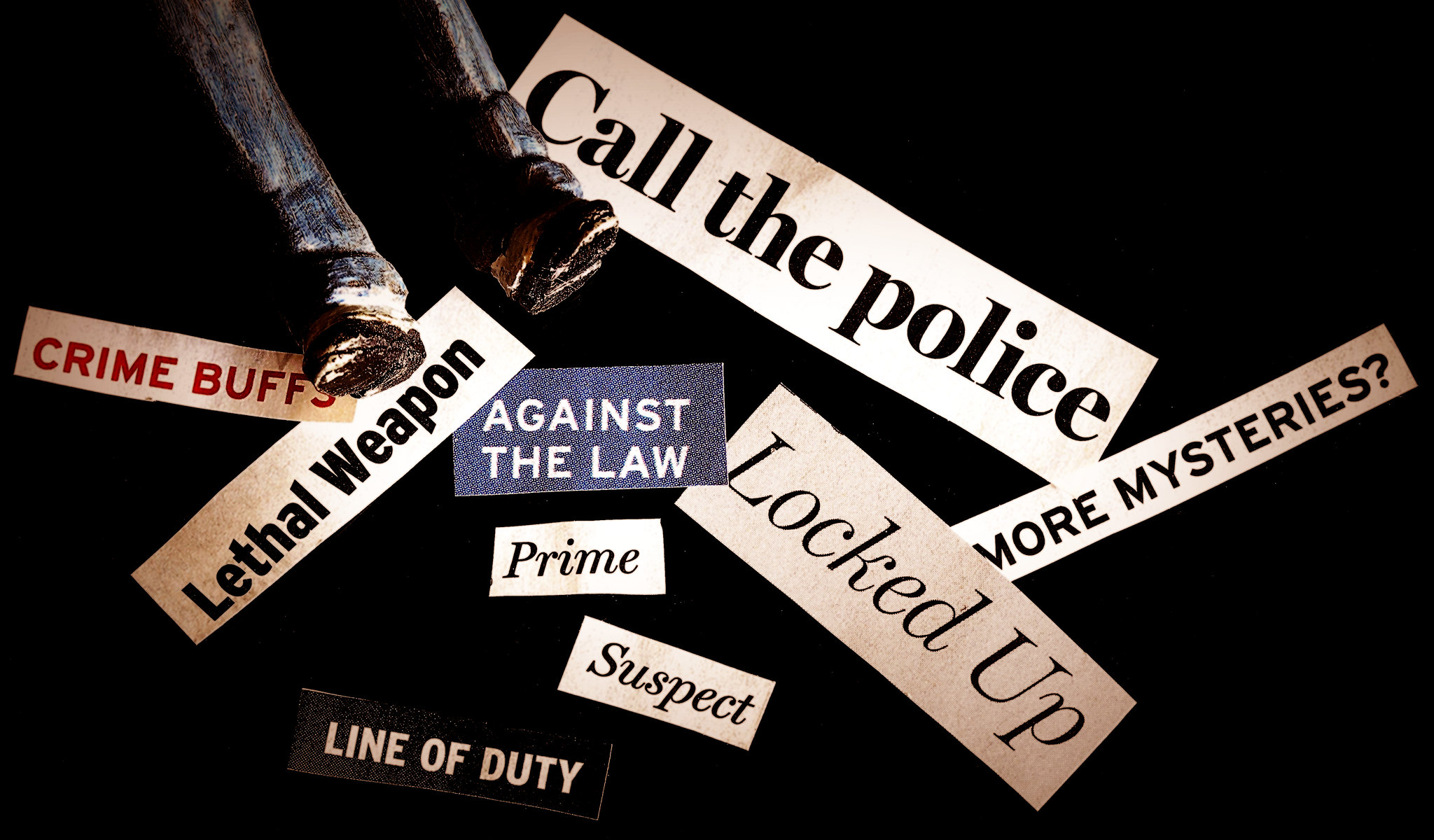This image features a dark, black background overlaid with various rectangular cutouts of titles and phrases, appearing to be sourced from newspapers or magazines. In the upper left corner, there are the legs of a mannequin or model, dressed in blue jeans and black tennis shoes, positioned as if suggesting the figure is in trouble or potentially injured. The words and phrases are scattered around these legs, creating a chaotic and ominous scene. Key phrases include "crime buffs" written in red capital letters with a white background, "lethal weapon" displayed diagonally in black font on white, and "call the police" positioned by the left foot in black font on a white rectangle. Other phrases such as "against the law" on a blue background with white font, and "prime", "suspect", "line of duty", "locked up", and "more mysteries" appear beneath or between the legs. Each phrase's design varies, with most having a white background and black font, yet others use distinctive color schemes, contributing to the overall collage effect on the stark black canvas.